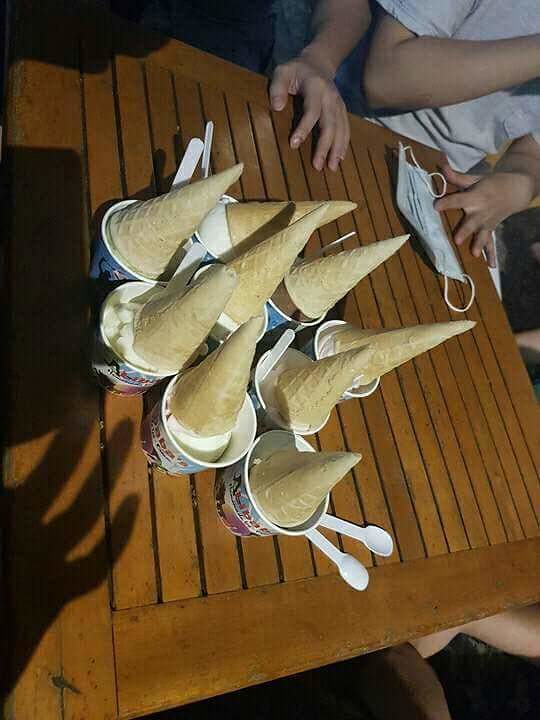The image is a detailed, overhead photograph of a wooden table surrounded by several people, with only their hands and parts of their arms visible. The table, made of medium brown slatted wood, displays nine small, white plastic cups, each with pink and purple writing that’s mostly obscured. Inside the cups, vanilla ice cream is topped with inverted waffle cones, creating a playful, upside-down effect. Scattered around the cups are several white plastic spoons, with some also placed in the cups. A light blue surgical mask lies beside one of the hands, contributing a modern and relatable detail. The people around the table, including a person wearing a white shirt visible at the forefront and another in a grey top, add a sense of liveliness and engagement to the scene. On the bottom left of the image, a hand shadow, presumably of the person taking the picture, falls across the table, adding depth and a hint of action to the composition. Overall, the photograph captures a moment of shared enjoyment and anticipation, possibly at an outdoor or patio setting.